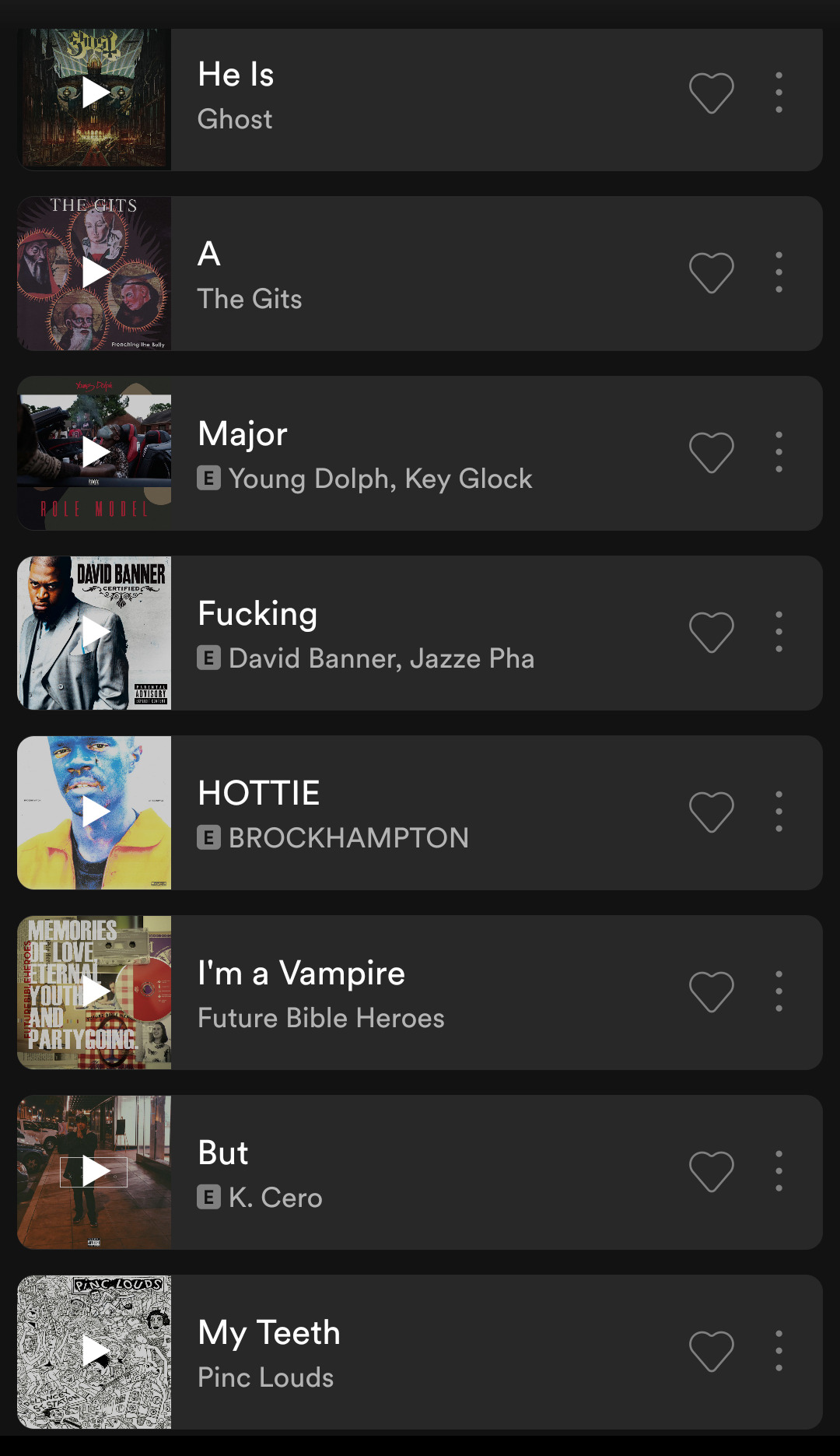The image showcases a music app in dark mode, characterized by its sleek design with white or grey text against a dark background. The screen features a list of various albums and their respective artists, with an interesting mix of genres prominently displayed, including metal and hip hop. The albums listed include:

- "He Is" by Ghost
- "A" by The Gits (G-I-T-S)
- "Major" by Young Dolph and Key Glock
- "Fucking" by David Banner
- "Hottie" by Brockhampton
- "I'm a Vampire" by Future Bible Heroes
- "But" by K. Cero (C-E-R-O)
- "My Teeth" by Pink Louds (P-I-N-C-L-O-U-D-S)

Each album entry features a play button on the album cover, which likely starts auto-playing the first track upon selection. There are also heart icons for users to like their favorite albums, along with additional options available to the right of each entry. The overall layout is straightforward and minimalistic, focusing on functionality without unnecessary embellishments. The combination of different genres adds an intriguing variety to the selection, catering to diverse musical tastes.